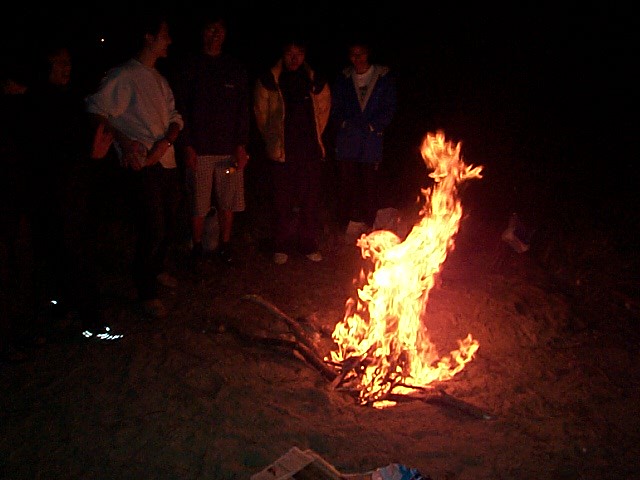In this nighttime outdoor photograph, a vibrant beach bonfire takes center stage, its flames roaring up to five feet high in vivid hues of orange and yellow. The fire consumes a pile of sticks, creating a striking contrast against the dark, sandy surroundings. Clustered dimly in the background are several people, their figures blurred and details obscured by the dark, but they seem to be enjoying the fire's warm light. One person, partially illuminated by the glow of a cell phone, leans forward, while others stand nearby, possibly wearing jackets and long-sleeved shirts. The scene is carefully captured with clear separation between the intense colors of the flames and the nighttime darkness, allowing for distinct visibility of the elements despite the low light. To the bottom left of the image, a series of small white lights, which could be from cell phones or other sources, shimmer faintly. The top right corner fades into complete darkness, adding to the overall mysterious and intimate atmosphere of the gathering.